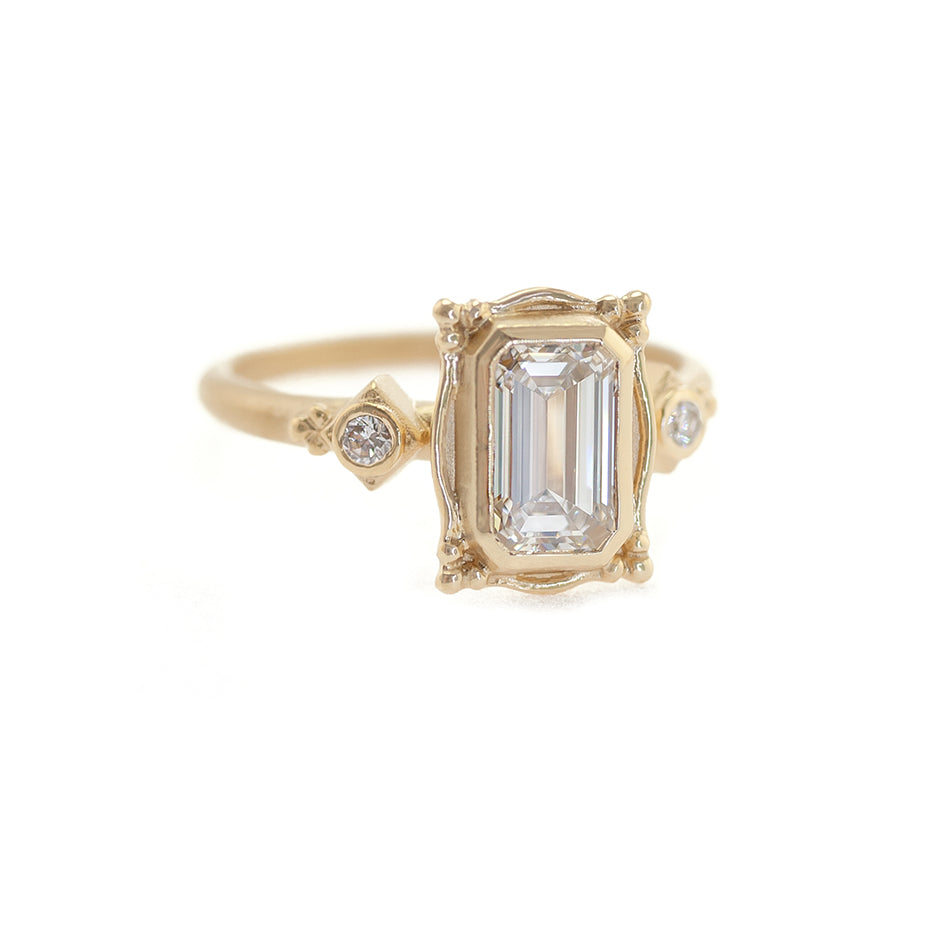This photograph showcases an elegant, premium gold ring set against a white background. The ring features a slender, understated gold band that transitions into an intricately designed top. The band, though simple, leads up to two smaller circular settings adorned with tiny, sparkling diamonds. Central to the design is a larger, square-shaped frame that houses a prominent, transparent, and reflective gemstone, likely a diamond, which exudes a brilliant shine. Additionally, elements of silver accentuate the design, framing the centerpiece and adding refined detail to the overall look, making this piece of jewelry exquisitely luxurious and visually captivating.